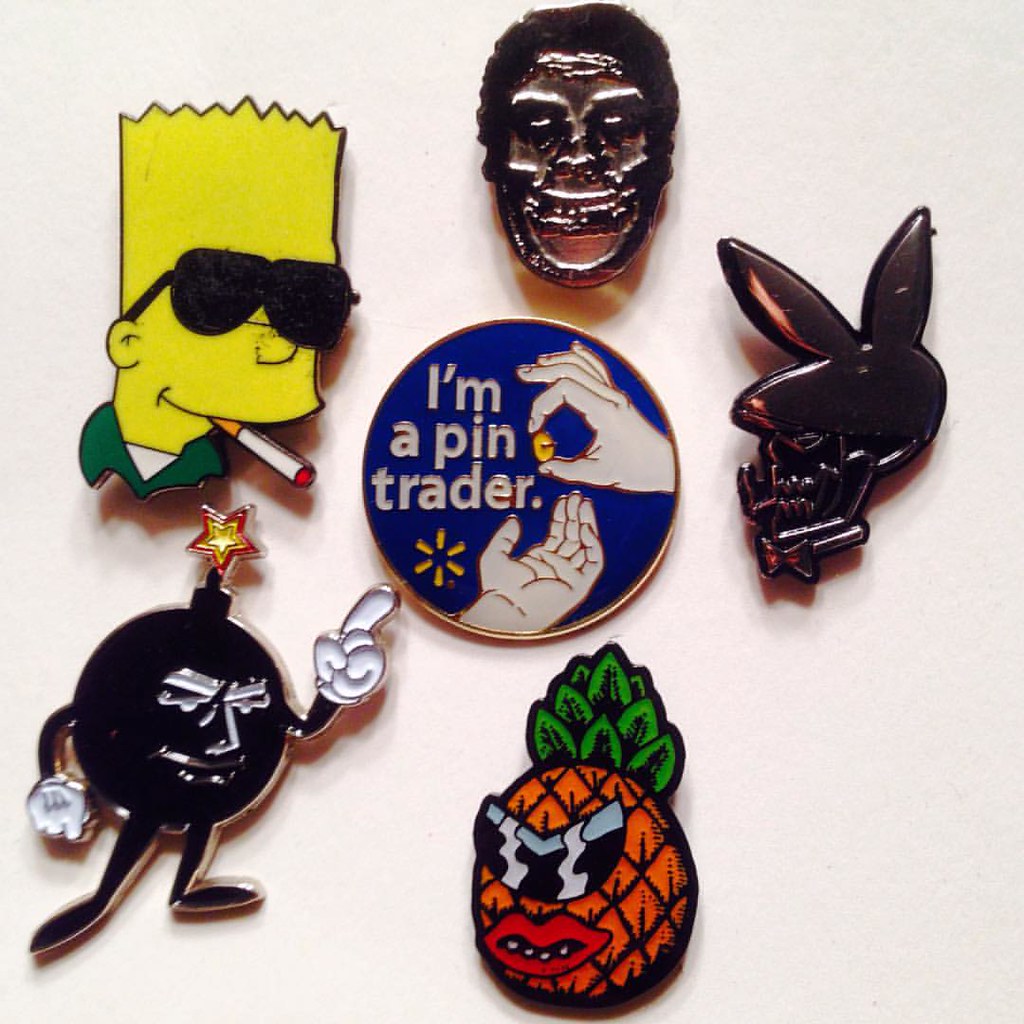In a square color photograph, displayed on a pink or light beige background, six collectible pins are neatly arranged in the center. The first pin features Bart Simpson wearing sunglasses and smoking a cigarette. Another pin resembles a cartoonish bomb with a face, hands, and feet, shaking its finger. There's also a pin shaped like an orange pineapple adorned with sunglasses and red lips. A blue circular pin stands out with the text "I'm a pin trader," showing an image of one hand handing a pin to another. Also included is a distinctive black pin that appears to mimic the Playboy bunny logo. Lastly, there is a pin that resembles a skeletal face. This visually engaging photo, likely snapped with a cellphone, captures an eclectic assortment of decorative pins perfect for adorning clothing or hats.